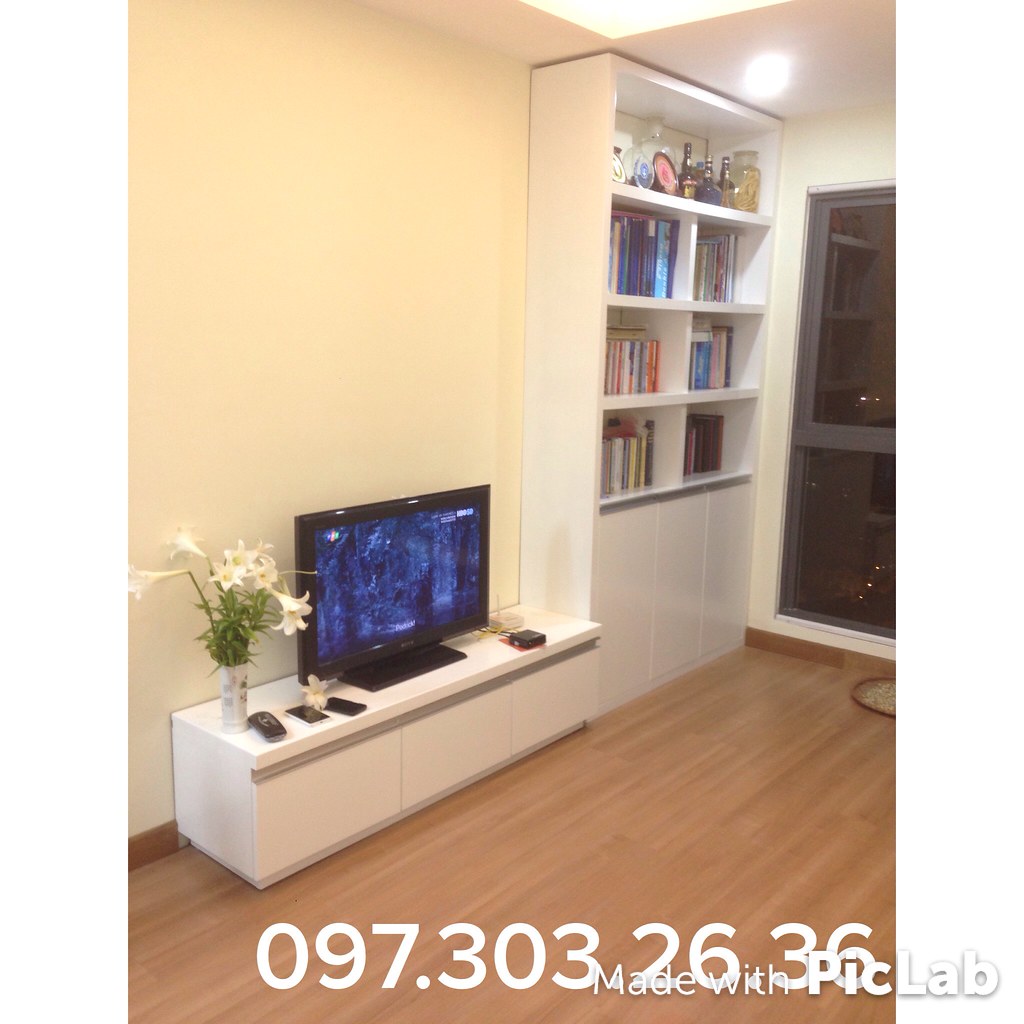The photograph captures the interior of a living room with a white ceiling, beige walls, and light brown wooden floors. On the upper left side of the image, there's a low white TV stand with gray trim, holding a small black flat-screen TV displaying a forest image. Beside the TV on the left, a vase filled with white lilies and green leaves stands tall behind a lineup of remote controls. On the right side of the stand, there are a couple of small objects, one black and square, the other white. 

To the right of the TV stand is a tall, white bookshelf with gray trim, featuring two columns of shelves. The top shelf holds various vases and glassware, while the other shelves are stocked with books. A large window on the right wall appears pitch black, suggesting it is nighttime. Below, the scene is anchored with light brown wood tile flooring. Additionally, bold white numbers, "097.303.26.36", and a "made with PicLab" watermark are visible at the bottom of the image.